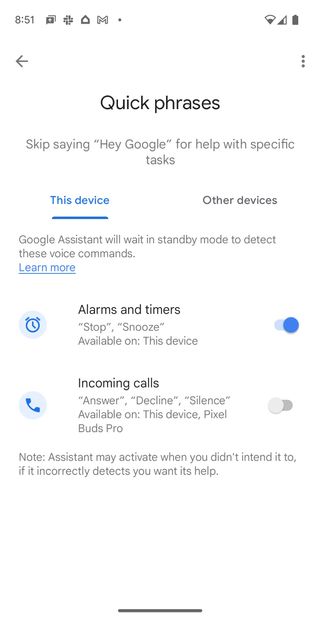A screenshot of a smartphone screen displaying various settings and options is observed. At the top-left corner, the time is shown as 8:51. To the right corner, the phone's status icons are visible, indicating a full battery and a decent internet connection. 

In the menu bar underneath, there is a back arrow to the left and three dots to the right, which suggest additional options when tapped. The main content of the screen appears to be a settings page for "Quick Phrases," which allows users to bypass saying "Hey Google" to execute specific tasks seamlessly.

The interface provides a toggle option highlighted in blue for enabling this feature on the current device and in gray for other devices. The description clarifies that Google Assistant will stay in standby mode to detect these voice commands without the wake-up phrase. A clickable link is also available to learn more about this feature.

Below this, the settings for alarms and timers are presented with a darker gray or black icon. The options "Stop" and "Snooze" are specified to be available on the device, with a toggle button, which is currently turned off.

Further down, an icon for incoming calls illustrates options to answer, decline, or silence calls available on both the device and PixelBread Pro. This setting is also turned off.

At the bottom of the screen, there's a noted disclaimer stating that the assistant may occasionally activate unintentionally if it incorrectly detects a need for its help.